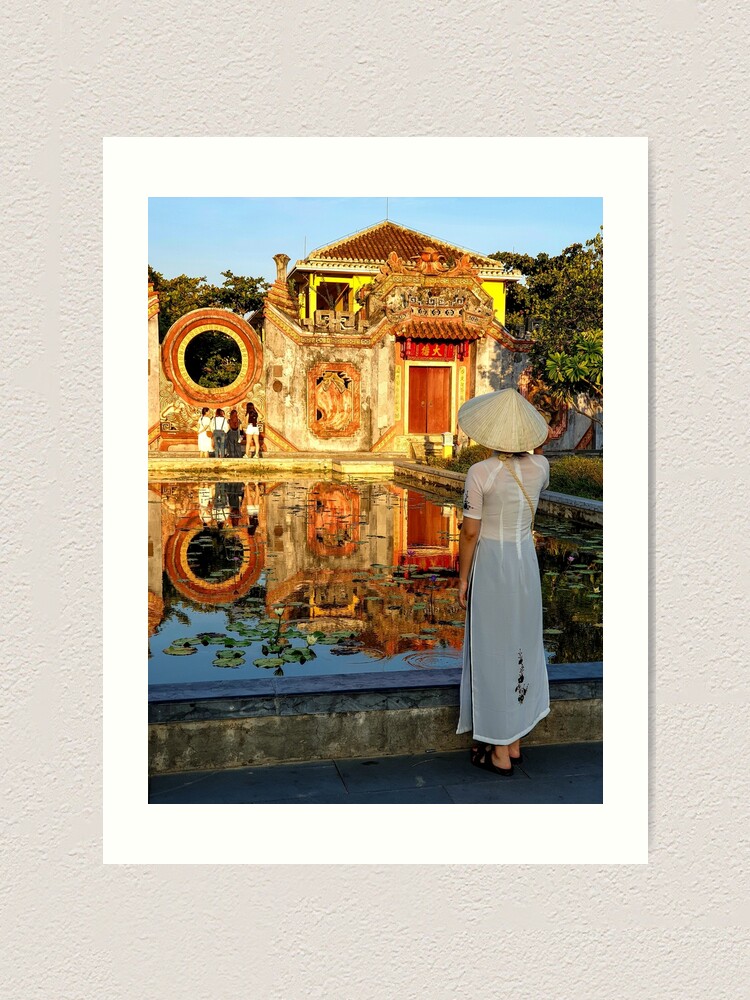The image is a vertically aligned rectangular picture, set against an off-white, textured background. At the center hangs a framed photograph with a thick white cardboard border. The photograph captures a serene scene under a bright blue sky. 

In the foreground, a woman stands with her back to the viewer. She wears an elegant, white lacy dress and a large, round beige-colored hat with a pointed tip. She appears poised and graceful as she gazes towards a temple-like structure, suggesting hints of Chinese or possibly Vietnamese architecture. This structure is painted in sunny shades of yellow and brown, with decorative elements including a circular cut-out on the left side where a group of young people stand. Some Chinese writing adorns the doors of this two-story building, which features a brown door and a yellow decorative piece above it.

The scene is set near a body of water dotted with lily pads, and the reflections of the group and the building add a layer of tranquility. Behind the temple, lush trees stretch towards the bright daylight sky, enhancing the overall peaceful ambiance of the image.